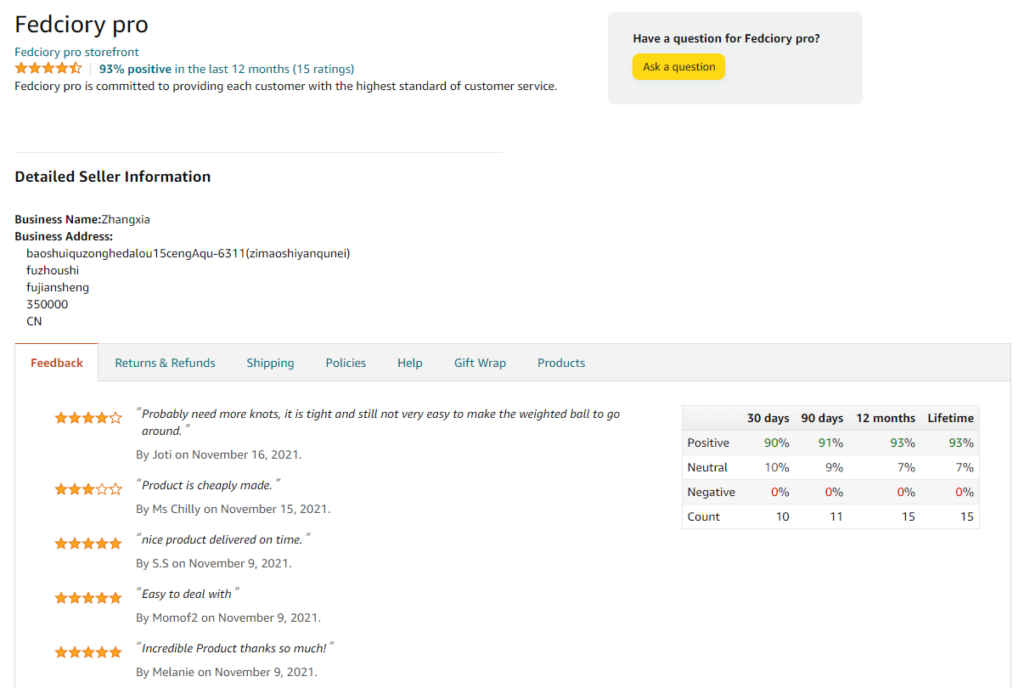**Detailed Description of the FedSiri Pro Amazon Storefront**

This image is a detailed screenshot of the Amazon web page for the seller FedSiri Pro. The storefront boasts a 93% positive rating over the last 12 months, based on 15 ratings. To visually depict this performance, there is a row of five stars where four and a half stars are highlighted in yellow to the left of the rating percentage. Below the ratings, a statement in black text reads: "FedSiri Pro is committed to providing each customer with the highest standard of customer service."

In the upper right section of the screenshot, encased in a gray box, there's text that says, "Have a question for FedSiri Pro?" followed by a clickable yellow button labeled "Ask a question" in black text.

Below this area is a thin horizontal gray line that spans about half the width of the page, under which is the heading "Detailed Seller Information." This section contains the business details such as the seller's business name, "Zangziya," and a somewhat unclear address: "15CNG-6311 in Ximei, Xiqui, Fuzhikui, Feng Shui," followed by another string of text "Line 35, 0000 CN."

At the bottom of the screenshot is a table displaying different types of feedback for FedSiri Pro. The headers in this table include Feedback, Refunds and Returns, Shipping Policies, Help, Gift Wrap, and Products. Under the highlighted Feedback section, five customer reviews are shown, each accompanied by star ratings:

1. **4 of 5 stars** - "Probably not, probably need more knots. It is tight and not very easy to make a weighted ball go around," by Jody on November 16th, 2021.
2. **3 of 5 stars** - "Product is cheaply made," by Miss Chili on November 15th, 2021.
3. **5 of 5 stars** - "Nice product, delivered on time," by SS on November 9th, 2021.
4. **5 of 5 stars** - "Easy to deal with," by Momof on November 9th, 2021.
5. **5 of 5 stars** - "Incredible product, thanks so much!" by Melanie on November 9th, 2021.

To the upper right of the Feedback table, there is a breakdown of positive, negative, and neutral ratings for various timeframes: the last 30 days, 90 days, 12 months, and lifetime. For these periods, the counts are as follows: 10, 11, 15, and 15 total ratings, respectively. The corresponding percentages for positive, neutral, and negative feedback are 90%, 91%, 93%, and 93%; 10%, 9%, 7%, and 7%; and 0%, 0%, 0%, and 0%. These percentages are visually distinguished by green text for positive ratings and red text for negative ratings.